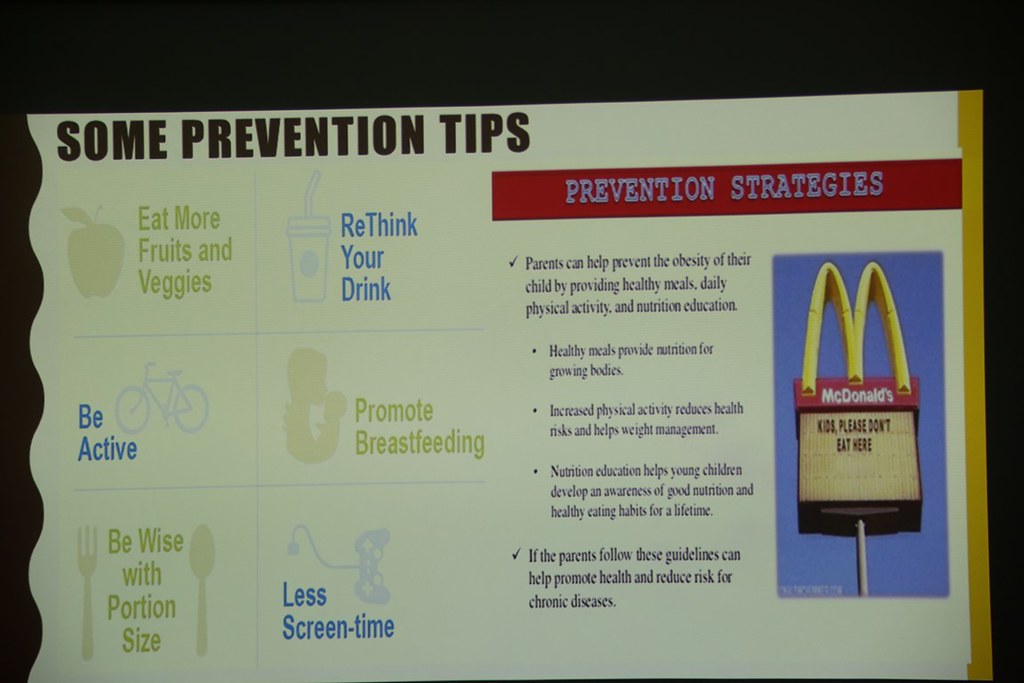The image features an educational poster centrally positioned against a solid black background. The background has a solid black field with a distinctive wavy black area on the left. The poster, with an off-white to grayish background, details various prevention strategies aimed at promoting child health. At the top left corner, bold black text reads "Some Prevention Tips," followed by illustrations and corresponding advice divided into two columns. The left column includes an apple saying "Eat more fruits and veggies" in green, a drink with a straw saying "Rethink your drink" in blue, and a bicycle saying "Be active," also in blue. The right column has a mother and baby labeled "Promote breastfeeding" in green, a fork and spoon saying "Be wise with portion size" in green, and an unplugged video game controller saying "Less screen time" in blue.

On the right half of the poster, a red horizontal banner reads "Prevention Strategies." Below this, bullet points elaborate that parents can help prevent childhood obesity through healthy meals, daily physical activity, and nutrition education. Benefits listed include providing necessary nutrition, reducing health risks, and promoting lifelong healthy eating habits. To the right of these paragraphs is a photo of McDonald's golden arches against a blue background, with a caption beneath urging kids not to eat there. The poster combines photographic representationalism and realism, employing colors black, tan, green, blue, yellow, and gray, making it both informative and visually engaging.